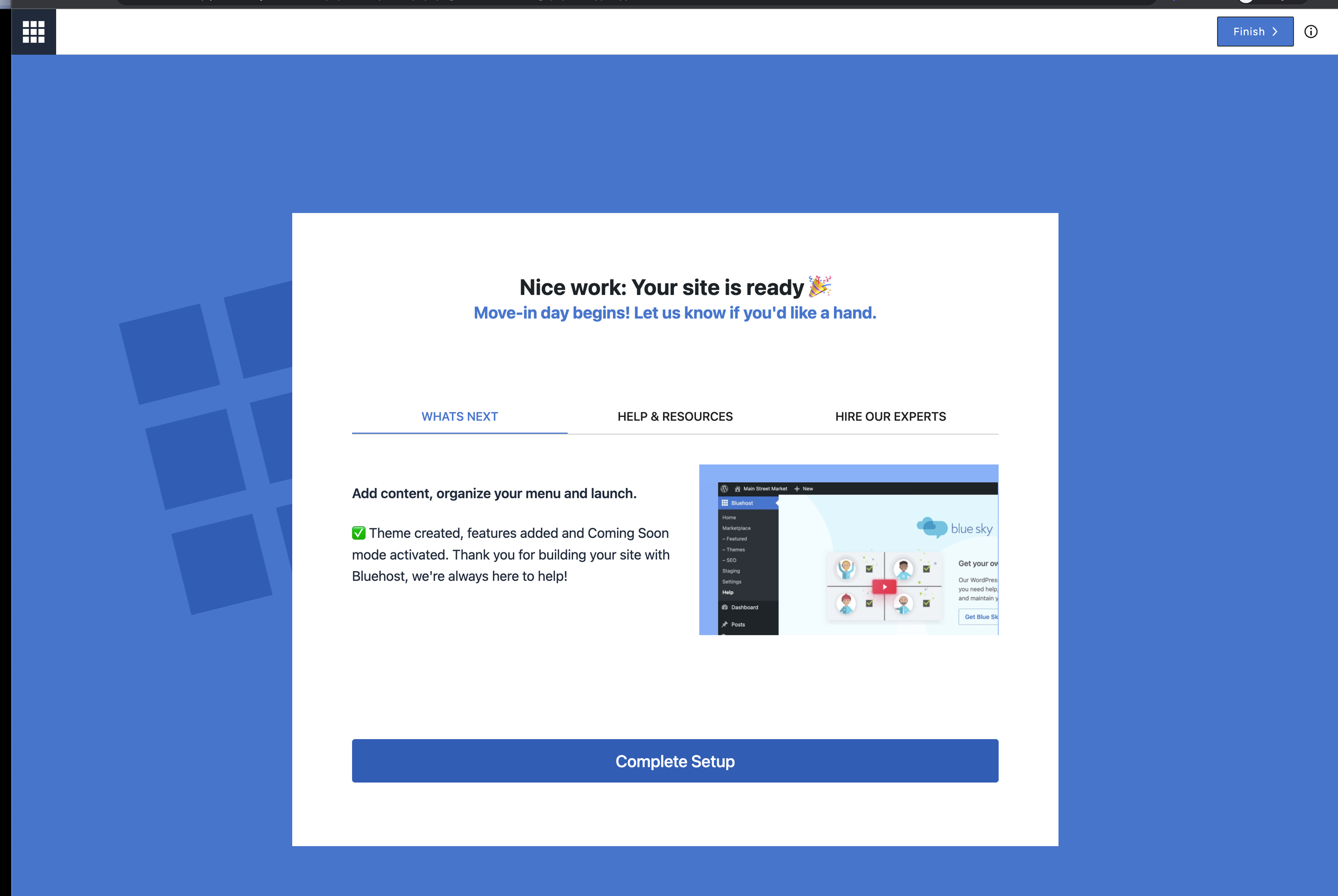This image showcases a webpage with a distinct layout and elements indicating the completion of a setup process. At the top, there's a border featuring nine squares forming a single square, accompanied by a "Finish" button with a right-facing arrow and an information icon on the far right. 

The main section of the page has a blue background, possibly portraying window-like sections. Prominently displayed is a pop-up notification congratulating the user with the message: "Nice work, your site is ready," adorned with a party popper icon. Below this, another message reads: "Move-in day begins! Let us know if you'd like a hand." 

Beneath the pop-up, there are three tabs: "What's New" (highlighted), "Help & Resources," and "Hooray from Our Experts." The subsequent text advises the user to "Add content, organize your menu, and launch." A checklist follows, indicating "Theme created" and "Features added" in a green box, with "Coming soon: Mode activated."

The footer of the pop-up provides a message of gratitude: "Thank you for building your site with Bluehost, we're always here to help." At the bottom of the screen, there is a "Complete Setup" button, ready for the user to finalize the process.